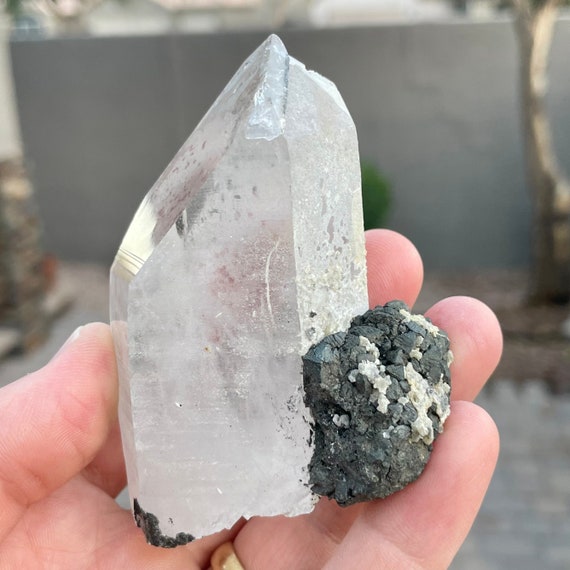In this detailed photograph, we see a close-up of a Caucasian male's left hand, partially visible from the bottom left corner, with a gold wedding band on the ring finger. His fingers delicately hold a large, white, translucent crystal that resembles a clouded rectangular prism, akin to the tip of a blunt sword with the top left facet slightly chopped off. The crystal, about the size of his palm, features a gray and white mineral growth roughly the size of a peach pit. Additionally, his hand grips another mineral to the bottom right—a smaller, dark, opaque rock that may resemble fool's gold, speckled with a few white spots. The background of the image is softly blurred, revealing hints of a light gray surface, a brown tree trunk to the right, and what appears to be a stone wall in the distance, contributing to a natural and earthy ambiance.